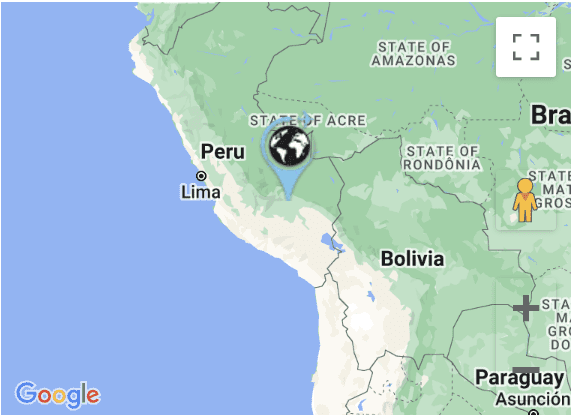This image depicts a Google Maps search highlighting a specific location in South America. The view is top-down, showcasing a broad swath of the continent, focusing particularly on Peru, Bolivia, and Paraguay. Notable features include the capitals and major cities such as Lima in Peru. Various regions such as the Amazon, Acre, and Rondônia are also highlighted.

To the left of the map, an expanse of ocean is visible, while the landmass of Peru is prominently featured on the right. A blue pin has been placed slightly east of Lima, centrally within Peru, marked with a small globe icon. Additional elements on the map include an orange figure, presumably the Google Street View mascot, which allows users to drop into street-level views, and an option to maximize the map view for an expanded perspective. The right edge of the image truncates neighboring countries.